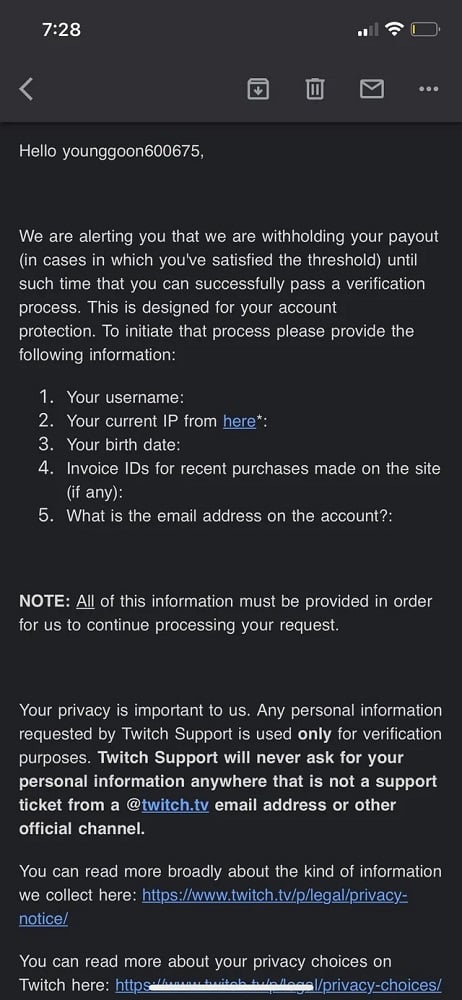A screenshot captured on a smartphone depicts an alert message from Twitch support. The background of the image is black, and on the upper left-hand corner of the screen in white text, the time is displayed as 7:28. Below the time, there is a white rectangle pointing towards the left, accompanied by a white envelope icon. At the top right corner, the battery icon indicates that the battery is low, showing a yellowish color.

The message reads: "Hello, younggoon600675. We are alerting you that we are withholding your payment. This is due to your account not yet satisfying the threshold to successfully pass the verification process. This measure is designed for your account protection."

Following this, the message provides instructions for initiating the verification process: "Please provide the following information:
1. Your username
2. Your current IP address (with 'here' underlined in blue)
3. Your birth date
4. Invoice IDs for recent purchases
5. The email address associated with your account

All of this information must be provided in order for us to continue processing your request. Your privacy is important to us. Any personal information requested by Twitch support is only used for verification purposes."